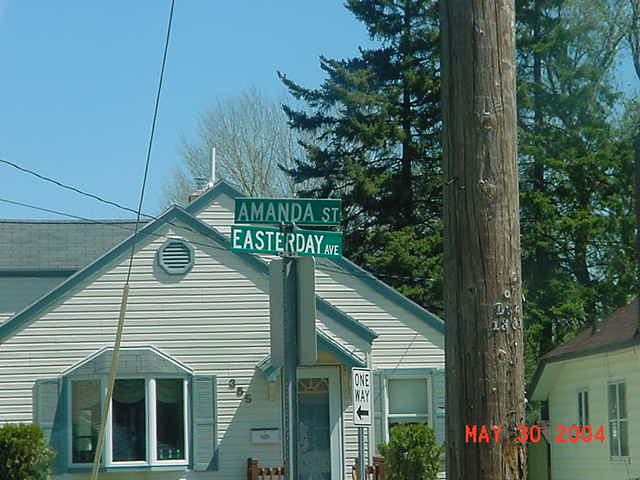The photograph, dated May 30, 2004, captures a street sign scene. Positioned on a metal pole, there are two signs: the top one slightly rotated but nearly flush with the bottom. The upper sign reads "Amanda Street," while the lower, a horizontal green and white rectangle, indicates "Easter Day Avenue." In the background, a charming one-story house features horizontal white siding and a bay window at the front. The front door, adorned with a storm door framed in white, holds a small mailbox attached to the house's exterior.